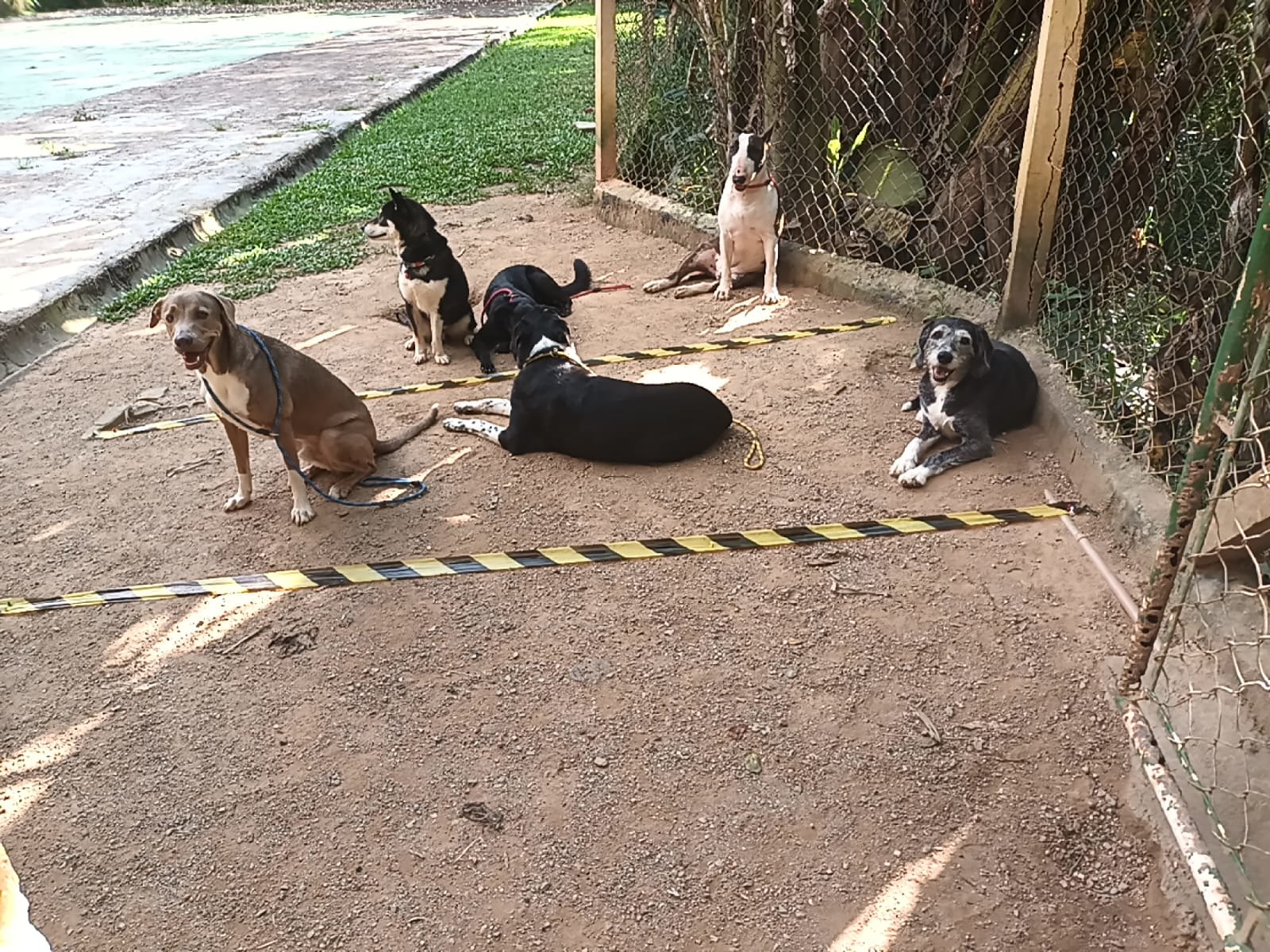This photograph captures six dogs resting together on a sandy dirt ground near a woven wire fence, backed by greenery and a parking lot. The ground is dotted with two pieces of caution tape lying between the dogs. The dogs vary in colors and postures: three are lying down and three are sitting. On the left, a grayish-brown dog with a white chest and forefeet wears a blue rope around his neck and is sitting while panting. Next, a black dog with speckled white paws and a white ring on his neck sports a yellow rope as he faces away from the camera. Nearby, a solid black dog adorned with a red rope lies on the ground. 

A striking black-and-white Husky with a white chest, muzzle, and legs is sitting and looking off to the right. Beside him, another dog with a white body and black markings around the eyes, ears, and tip of the nose is sitting sideways on his haunches, possibly equipped with a red collar. Finally, an elderly dark gray dog with a white muzzle, chest, and feet is lying down, facing the camera with his mouth open. Amidst them, a small Shiba Inu, black and tan in color, adds to the diverse mix. The scene is set against the backdrop of a dirt and gravel ground, framed by a fence supported by wooden posts.